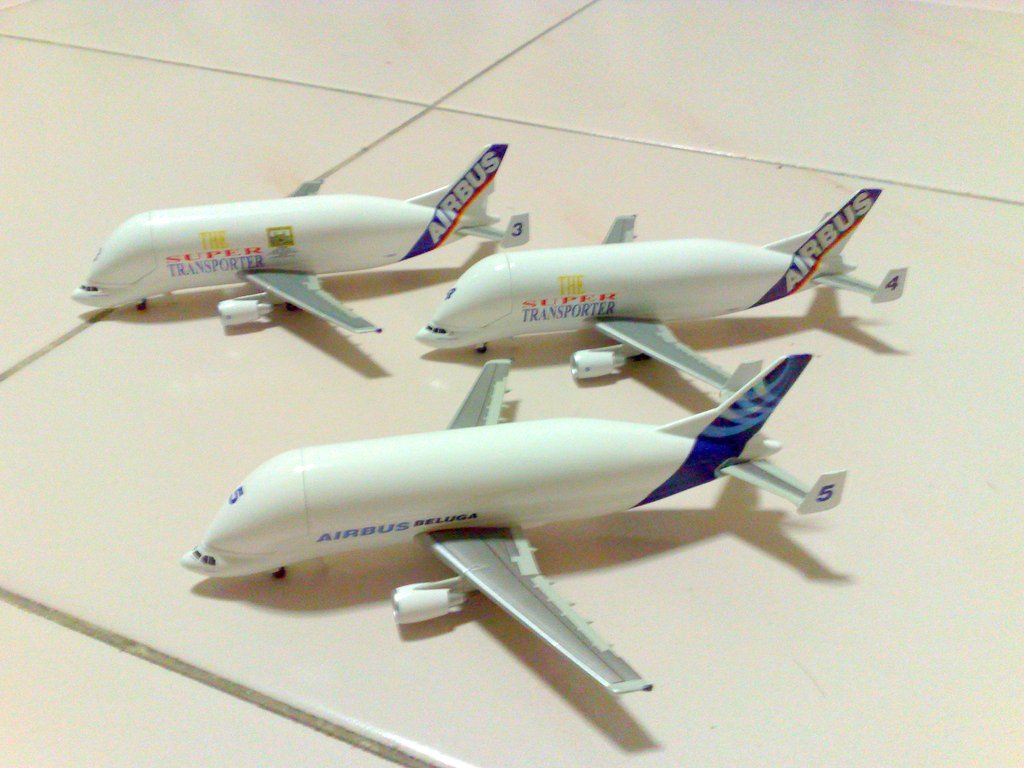The image captures a diagonal top-down view of a tiled floor, showcasing five large, off-white tiles with gray grout lines. Centered predominantly on a single tile are three model airplanes arranged in a formation resembling a backward-pointing triangle. The planes are distinctly reflective, appearing to be made from a plastic or rubber material, and all bear the Airbus logo. 

The two planes at the top of the image, each with gray wings, are virtually identical, both featuring the text "Transporter" and multicolored graphics, including red dots above the lettering. The left plane has a number 3 on its tail fin, while the right one has a number 4. Both have blue stripes interspersed with red on their tails and Airbus written in white. 

The third plane, positioned in the foreground and slightly larger, displays "Airbus Beluga" on its body. Its tail fin is marked with the number 5 and adorned with a dark blue, light blue, and gray swirl design. The body of this model is also white with blue graphics, distinct from the bright multi-colored designs on the other two. 

The photograph beautifully highlights the trio of detailed Airbus models against the contrasting light tiles and dark grout, creating a striking display.